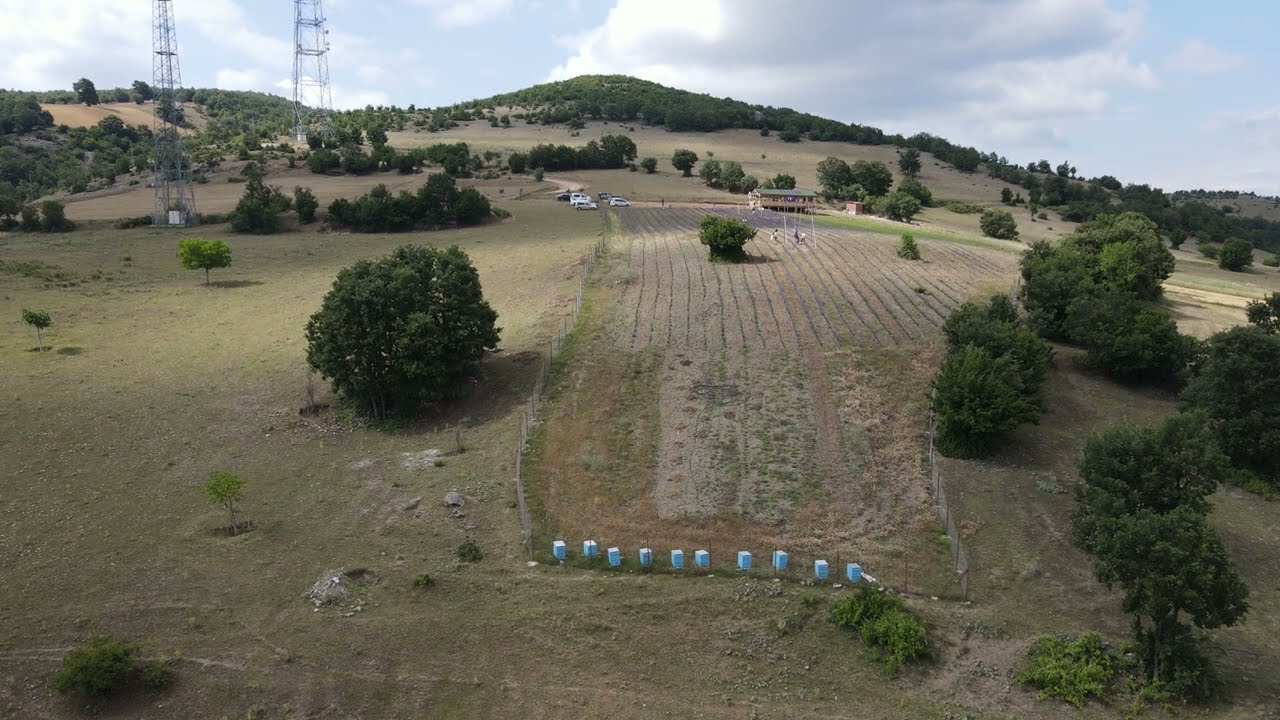This overhead photograph captures a vast, slightly hilly ground area predominantly covered in light green grass, creating a wavy texture. Scattered throughout the landscape are clusters of trees with dense groupings at the hills' peaks, contrasting with sparser regions. Central to the image is a rectangular tilled field with parallel vertical lines indicative of ploughing, possibly suggesting a farm. Flanking this area, several light blue rectangular items—potentially beehives—are arrayed in a rough row. Adjacent to this cultivated field is a house structure with vehicles parked nearby. On the left side, silver electrical towers rise against a backdrop of a blue, cloud-filled sky, blending agricultural and residential elements seamlessly.